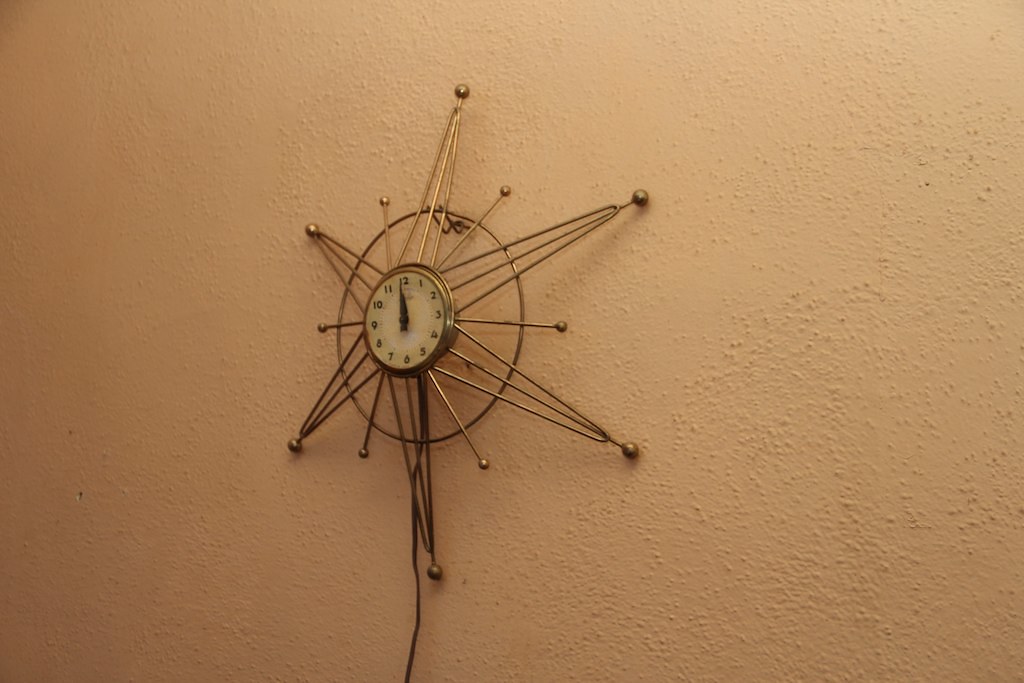The image depicts a textured beige wall, intentionally designed with a bumpy surface. Mounted on this wall is a striking clock with a unique star-shaped design. The clock features a circular metal frame with a star-like pattern, likely bronze in color, emanating from its center. Within this star pattern is a smaller circle that houses the clock face. The clock face itself displays the numbers 1 through 12 in a clear, black font. The hour and minute hands, also black, indicate that the time is a few minutes shy of either noon or midnight.